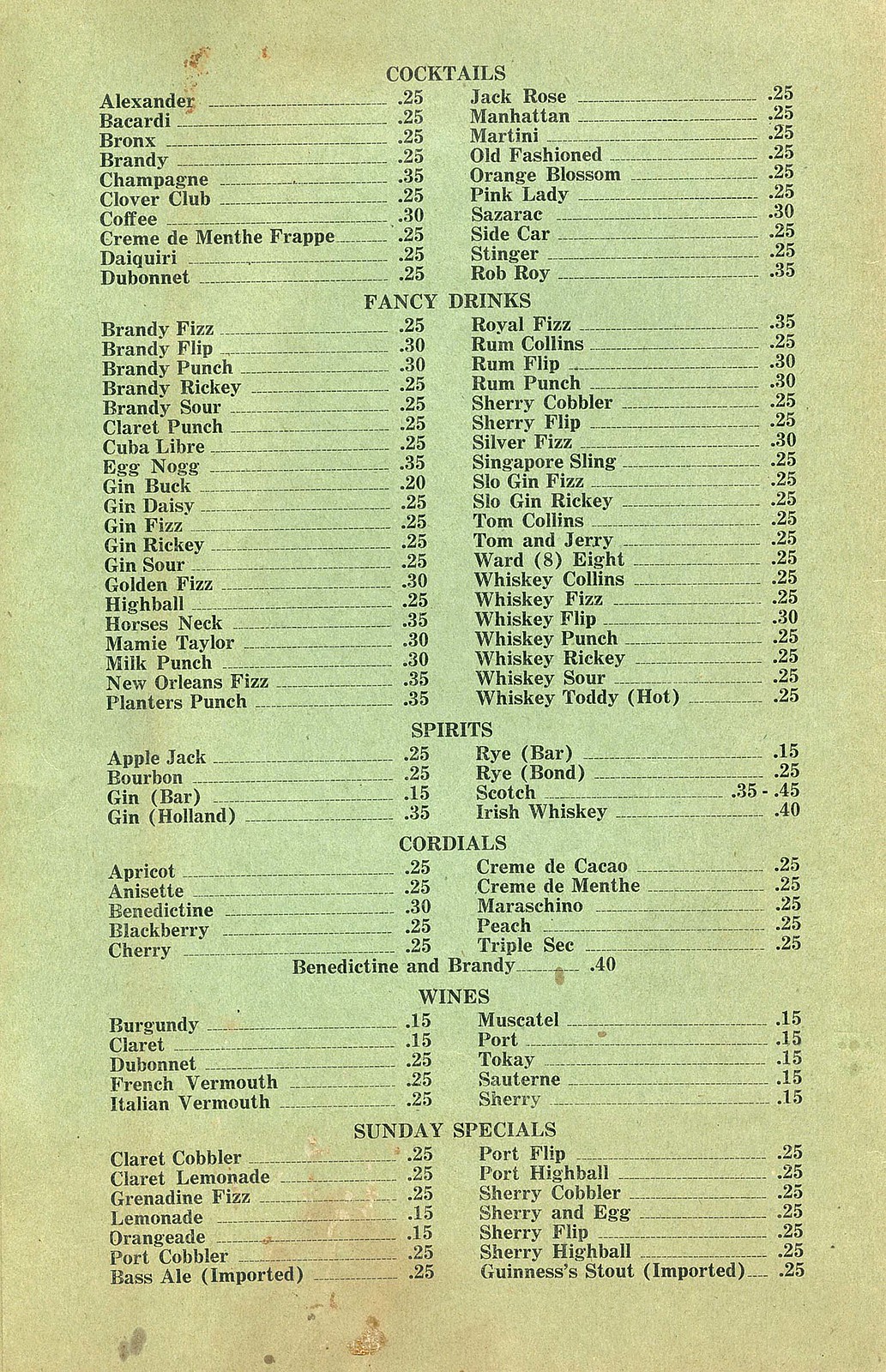This image captures a photograph of a rectangular drink menu, predominantly off-white in color with a notable large brown stain in the bottom middle. The menu is divided into six distinct sections, each meticulously itemizing beverages alongside their corresponding prices. 

At the top, the first section, labeled "Cocktails," features a variety of cocktail options, with each drink name aligned on the left and its price on the right. Directly below, the "Fancy Drinks" section similarly lists an array of names, each accompanied by its price on the right.

Continuing downward, the "Spirits" section stands out with a concise selection of eight spirits, each with its price to the right. Following this, the "Cordials" section presents a list of cordials, again with prices noted to their right. 

The penultimate section showcases an assortment of wines under the "Wine" heading, systematically listing each wine with its price adjacent on the right. Lastly, the "Sunday Specials" section rounds out the menu, offering specific drink options available on Sundays, with prices listed on the right. 

Overall, the menu's detailed organization and clear price listings provide a comprehensive guide for patrons to explore their beverage choices.